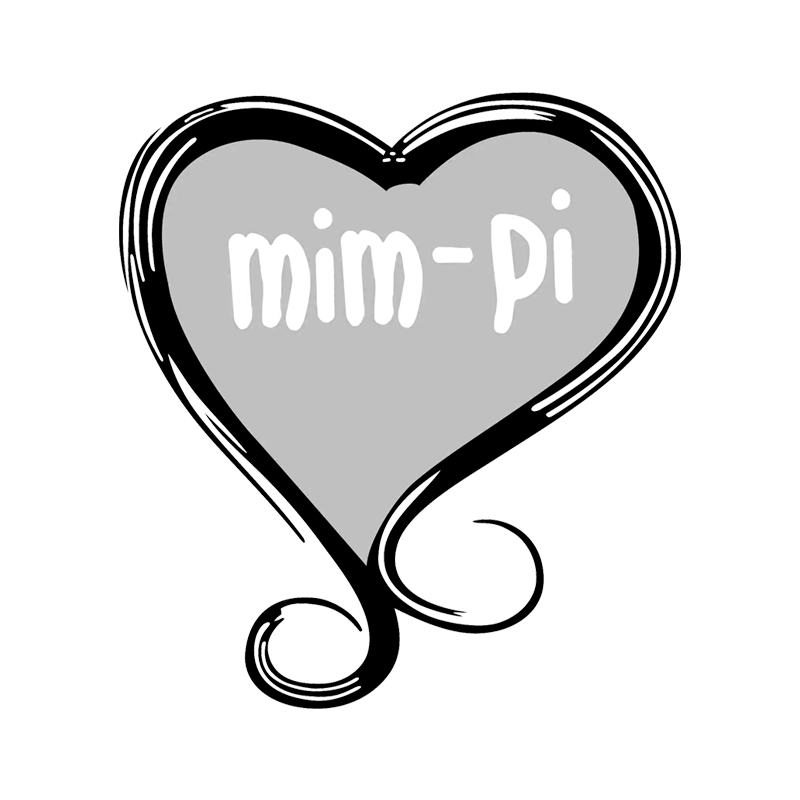The image features a black, white, and gray illustrated heart with a thick, sketchy outline and decorative curled ends on the left and right sides, resembling a stylized mustache at the bottom. Inside the heart, the center is filled with a light gray while the remainder is partially white. Across the heart, the word "MIMPI" is written in white, lowercase, bubbly letters. The heart is set against a plain white background, giving it a floating appearance.